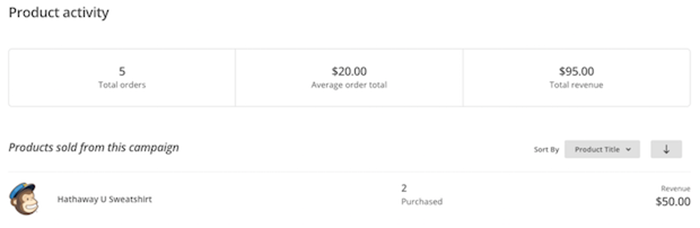**Detailed Caption:**
This image features a product activity screen, likely from MailChimp, as indicated by the recognizable MailChimp monkey logo adorned with a hat. At the top left, the header "Product Activity" is displayed prominently. The main section is divided into three distinct segments, each containing numerical data followed by descriptive text in light gray.

1. **Middle section:**
   - The first metric shows "5 Total Orders" in bold black text, with the accompanying text in a smaller light gray font stating the same.
   - The second section highlights an "Average Order Total" of $20.00, formatted similarly with the smaller descriptive text below.
   - The third segment presents the "Total Revenue" as $95.00, again following the same pattern of presentation.

2. **Lower Details:**
   - Below these metrics, there’s italicized black text on the left that reads “Product Sold From This Campaign.”
   - Adjacent to this section, "Hathaway U Sweatshirt" is listed as the product sold. Further details specify two units were purchased, generating a revenue of $50.00.

3. **Additional Features:**
   - To the right of the product details, there is a sort function labeled "Sort by Product Title" presented on a gray field with black text and a drop-down menu.
   - Adjacent to the sort function, a download button is displayed, signified by an arrow pointing downward.

4. **Background:**
   - The entire screen is set against a clean, white background.

Although the screen doesn’t explicitly state “MailChimp,” the presence of the familiar logo and the context suggests it's detailing the results of an email marketing campaign, highlighting the successful sales generated from the campaign.